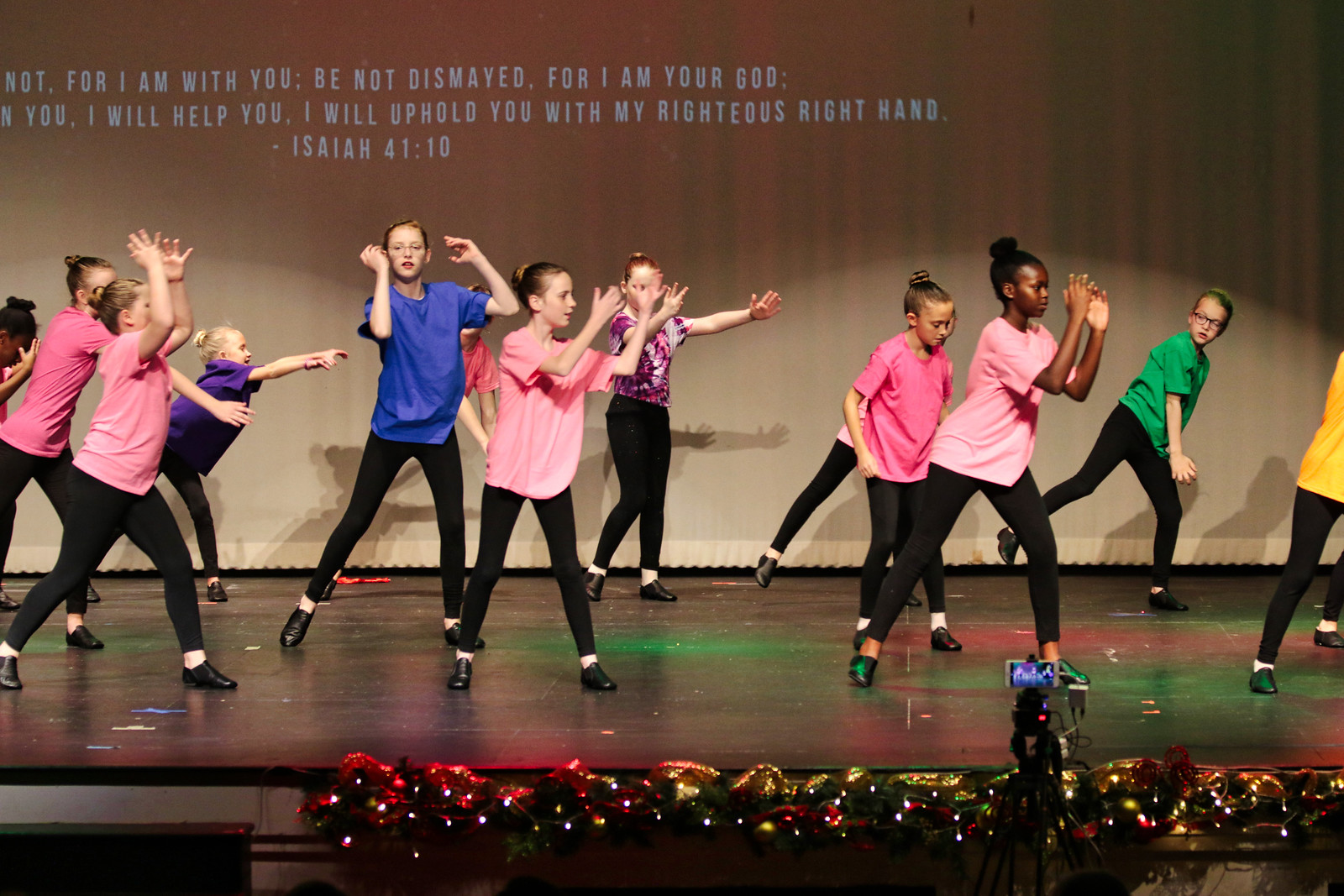In this photographic image, set indoors in a school auditorium, a group of children is gathered on a decorated stage, likely for a performance with a religious theme. The stage front is adorned with Christmas decorations, and bright lights illuminate the foreground. A camera is visible in the bottom right corner of the image, capturing the event.

In the center of the stage, a diverse group of children appears to be singing and dancing. Among them are mostly girls in their early teens, dressed in black pants and black sneakers. Their attire predominantly features pink short-sleeved shirts, worn by five of the girls. One girl is wearing yellow, another has a blue outfit with glasses, another wears purple, and yet another girl dons a tie-dye purple shirt. The children are mostly white, except for one black girl standing near the right side of the photo. Additionally, a white boy with glasses, dressed in a green shirt and black pants, is part of the group.

Text is displayed at the top left corner of the image, quoting Isaiah 41:10: "Not for I am with you, be not dismayed for I am your God. I will help you. I will uphold you with my righteous right hand." This suggests that the scene might be of a performance in a church or a Christian congregation’s event. The overall atmosphere conveys a spirited and inclusive celebration.